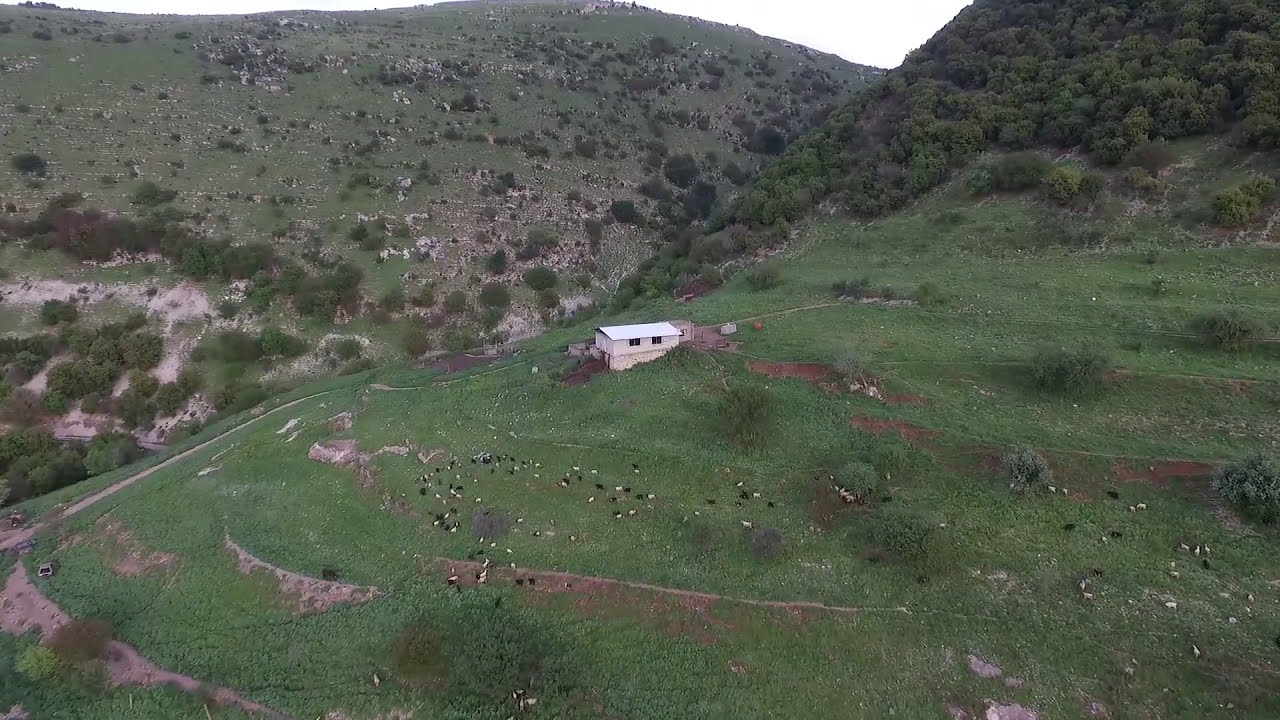This photograph captures an expansive, elevated view, likely taken from a high vantage point such as a drone or a mountaintop, showcasing a hilly terrain rich with detailed features. Central to the image is a white house, possibly a farmhouse or barn, standing amidst the lush greenery. The house has two visible windows and is notably situated on the lower side of a hill covered predominantly with grass. The upper portion of the hill is densely wooded, transitioning into a tree line that extends to the upper right-hand corner of the photo. In this verdant expanse, clusters of trees and bushes are interspersed, punctuating the grassy landscape.

In the foreground, a herd of cattle, numbering perhaps a hundred, can be seen grazing. The terrain features terraced levels with exposed brown soil visible through breaks in the grass. Beyond the central hill, another rises in the background, similarly adorned with grass and trees, though marked by patches of dry, brown areas.

To the left, the scene hints at a road or potentially a river, though it's distant and partially obscured. The surrounding field appears mostly barren aside from the grass, with minimal signs of human activity or infrastructure. The sky overhead is a uniform white, complementing the serene, natural setting depicted in this high-altitude shot.